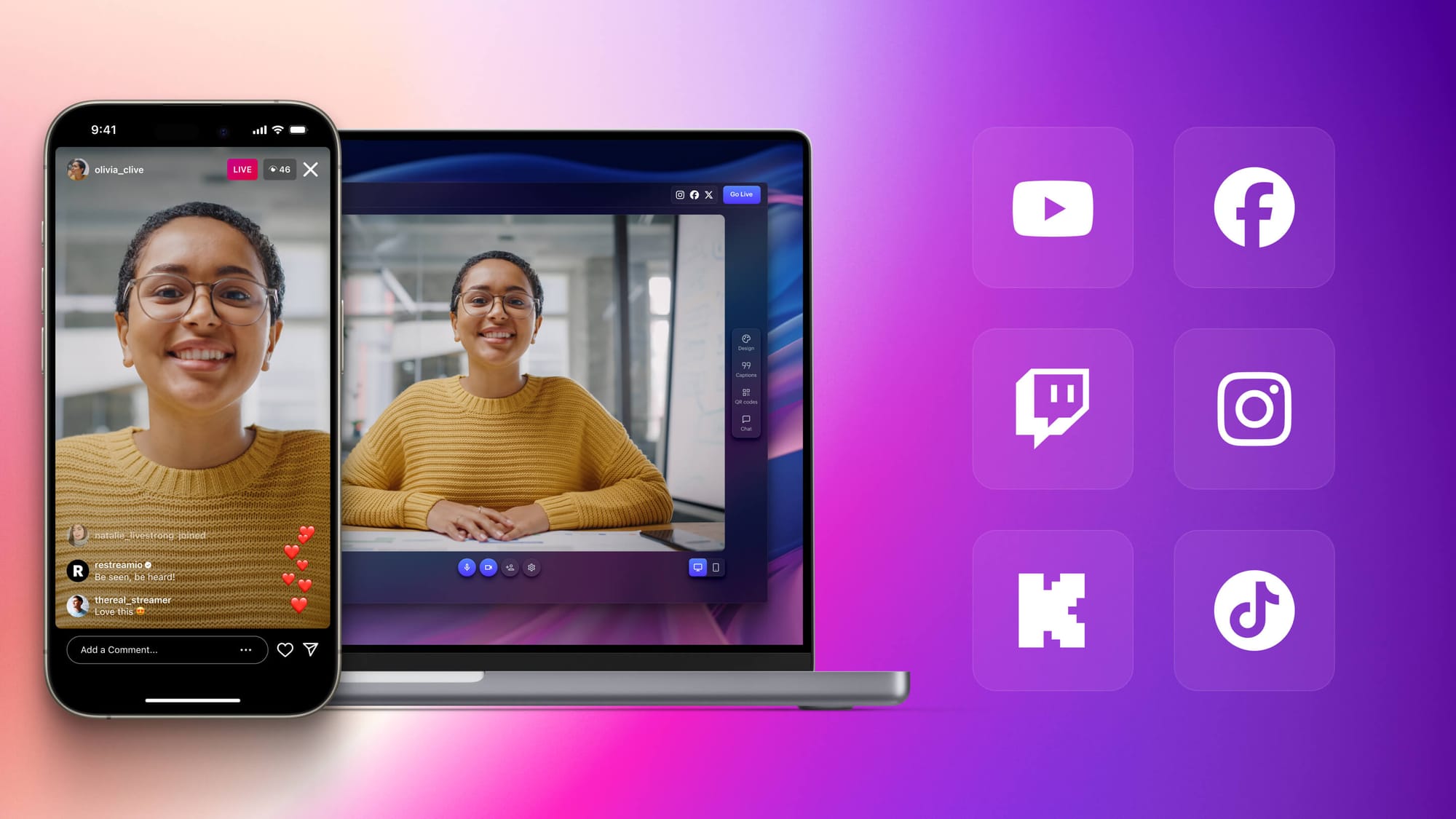The advertisement showcases an electronic company's devices, prominently featuring a landscape-oriented image with a gradient background that transitions from pink on the left to purple on the right. On the left side, a smartphone and a laptop are displayed, both showing the same woman actively participating in a video call. The woman, who is smiling, is wearing brown glasses and a dark yellow or goldish sweater, and has dark skin and black hair. The video call on the smartphone screen includes chat interactions and reactions, suggesting a dynamic conferencing environment. Overlaid on a purple background to the right are six app icons arranged in two rows of three, including recognizable logos for YouTube, Facebook, Instagram, TikTok, and two other unidentified social media platforms. The ad effectively highlights the integration and harmony of the company's smartphones and tablets with popular social media and video conferencing applications.